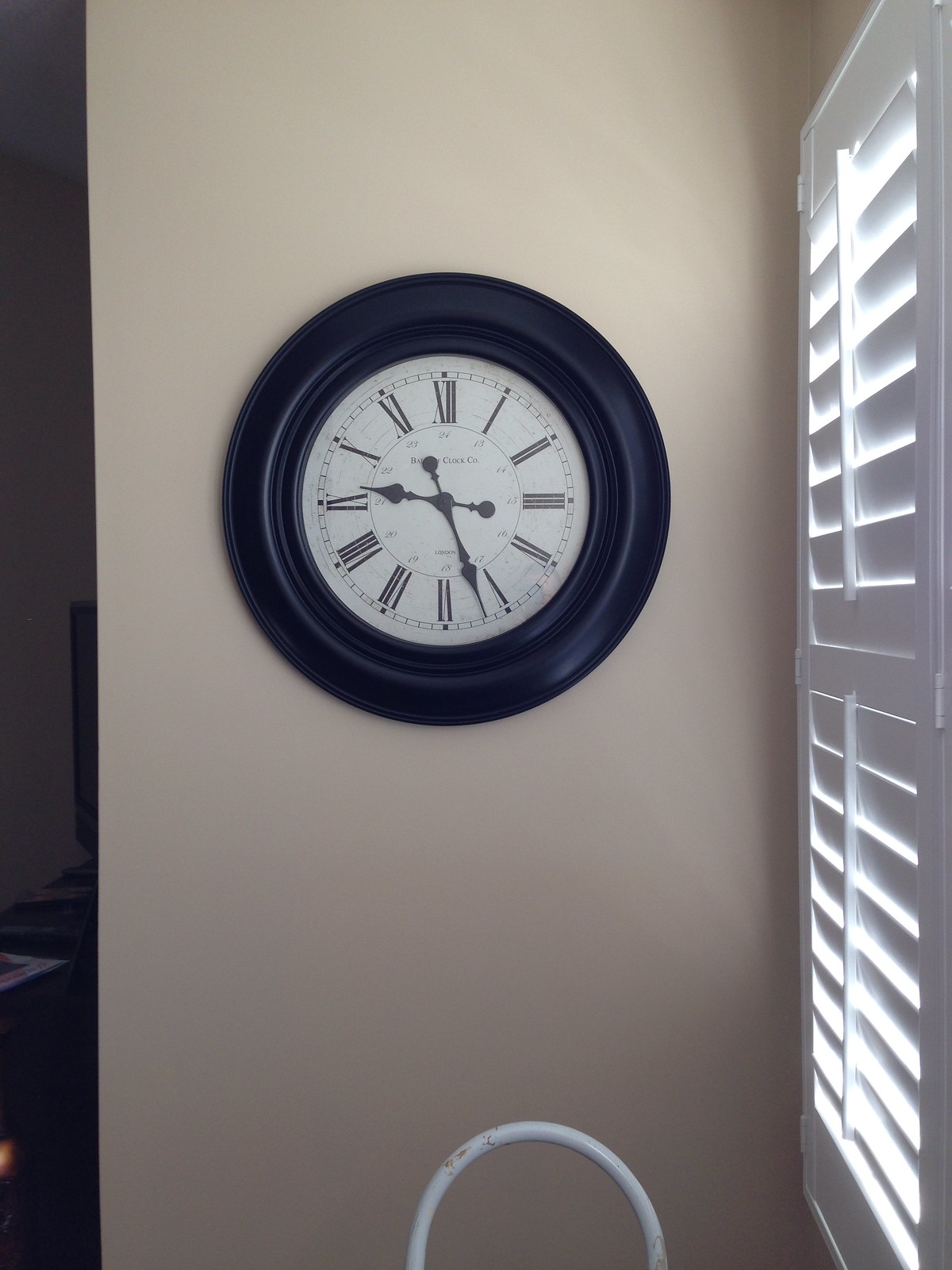A vertical photograph capturing a beautifully lit, cozy interior scene. At the center of the image is a wall adorned in a soothing, light taupe paint. Dominating the wall is an elegant clock, featuring a robust black frame that adds a striking contrast to the muted backdrop. The clock's face is marked by traditional numerals, lending a classic ambiance to the room. On the right side of the frame, white shutter blinds, partially open, allow gentle beams of sunlight to stream in, illuminating a segment of the clock and suggesting a serene daytime atmosphere within the home.